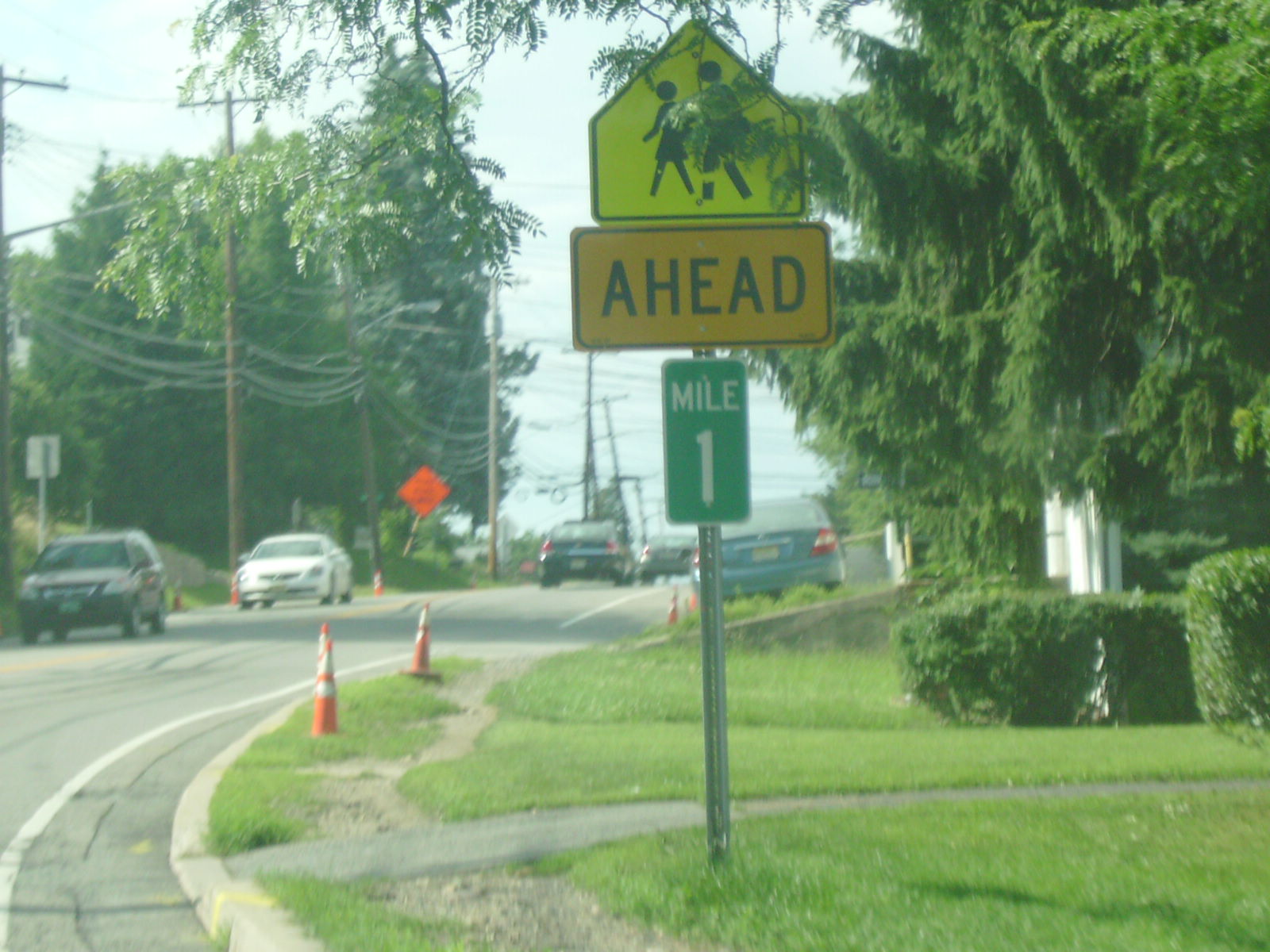This outdoor photograph captures a detailed streetscape where the focal point is a multi-sign post standing amidst the scene. The pole, planted in a grassy area, supports three distinct signs. At the top is a traditional school crossing sign shaped like a pentagon with a yellow background, black border, and a graphic of two people carrying books. This sign is partially obscured by foliage from a nearby evergreen tree. Below it, a horizontal, rectangular, yellow sign with "AHEAD" written in bold black letters also features a black border. The third sign is a vertically-oriented rectangular green sign with "MILE 1" in white letters.

In the lower part of the image, the street curves to the right, where several construction cones indicate ongoing road work. The scene shows two cars approaching and two cars driving away, with another car parked on the right side of the street. Additional orange construction cones are scattered near the vehicles, with an orange diamond-shaped "ROAD WORK AHEAD" sign adding context to the disruption. The presence of trees outlines the background, enriching the composition with natural elements.